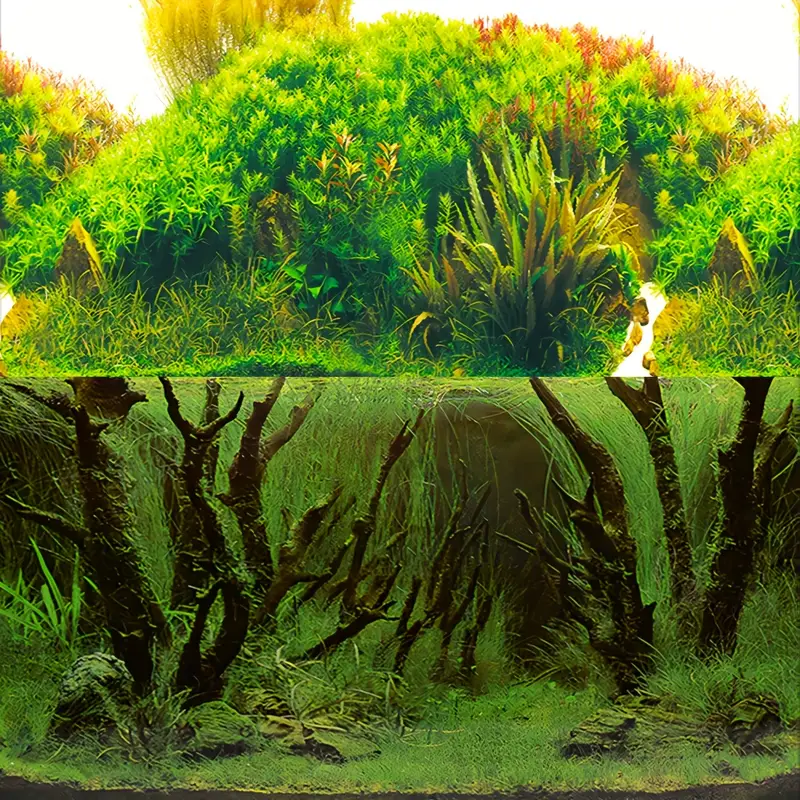The image showcases the interior of a sophisticated aquarium or terrarium, skillfully designed in an aquascaping style. The clear glass structure is filled with water up to halfway, creating a vivid visual interface between the submerged and aerial environments. Above the water, the scene features thriving green plants with some reddish-yellow touches, indicative of multiple plant species. The roots, reminiscent of wooden structures, are dark brown or black in color and dramatically delve beneath the water's surface.

Underwater, the setting is equally lush with green moss and grass-like growth. Small pebble-like rocks dot the ground, enhancing the natural aesthetics. The water-bound roots appear heavily encrusted with moss and intertwine with seaweed-like plants that sprout from the substrate. The terrestrial plants above flourish in what appears to be a sunny environment, with their large, pointed leaves basking in the clear light. Overall, the meticulously crafted setup harmonizes both aquatic and terrestrial elements, creating a cohesive ecosystem within the glass confines.